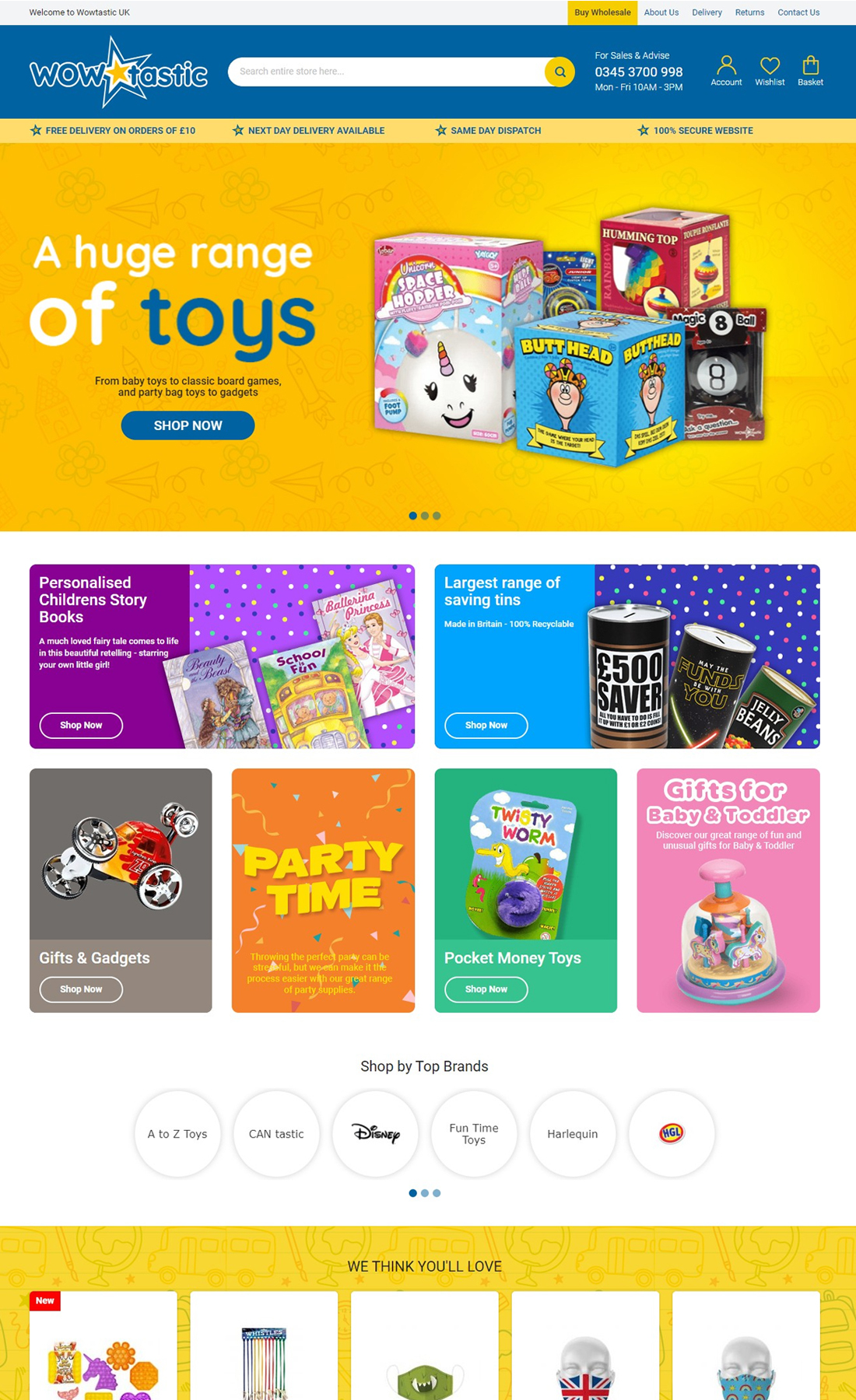Screenshot of a Kid's Toy Store Website:

At the top of the screen, there's a blue banner displaying the store's name "Wowtastic" with a yellow star situated between 'Wow' and 'Tastic.' Adjacent to the banner, there's a search bar equipped with a yellow search icon. To the right of the search bar, the contact information reads: "For sales and advice: 0345 370 0998," available Monday through Friday from 10 a.m. to 3 p.m.

Moving along, there are three icons for navigation: a person icon labeled "Account," a heart icon labeled "Wishlist," and a shopping bag icon labeled "Basket."

Below the blue banner is a yellow banner that includes additional offers and information. A blue star accompanied by blue text announces: "Free delivery on orders of £10," followed by "Next day delivery available," "Same day dispatch," and "100% secure website," all separated by stars.

The main part of the image features various toys. Prominently displayed is a toy named "Space Hopper," alongside "Butthead Humming Top," and the "Magic 8-Ball." To the left of these images, bold blue text states "Toys," preceded by "A huge range of" in white font. Below that, it reads: "From baby toys to classic board games and party bag toys to gadgets." There is a blue "Shop Now" button beneath these descriptions.

Further down, additional images of toys and categories are displayed with labels such as "Largest Range," "Saving Tens," "Profit Money Toys," "Party Time," and "Just for Baby and Toddler."